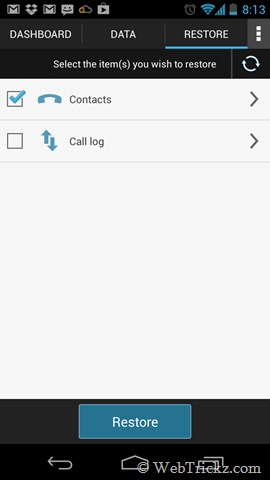This screenshot, taken on a mobile device, showcases a screen related to data restoration. The upper left-hand corner of the screen features several application icons. On the upper right, icons for an alarm clock, Wi-Fi connection, cellular service bars, a low battery indicator, and the current time displayed as 8:13 are visible. There are three tabs at the top labeled "Dashboard," "Data," and "Restore," with "Restore" selected and highlighted by a blue underline. Adjacent to the tabs, a menu represented by three vertical dots is visible.

Below these tabs, text instructs the user to "Select the items you wish to restore." Directly underneath this instruction, a refresh button is placed. The options "Contacts" and "Call log" are listed below, with a checkbox next to each option; "Contacts" is checked, whereas "Call log" is not. Both entries have arrows pointing to the right, suggesting further interaction.

A considerable blank space follows, leading to a prominent "Restore" button situated at the bottom of the screen against a black background. In the lower left corner, an arrow is pointing to the left, likely for navigation purposes. The lower right corner features the text "webtricks.com" in white font.